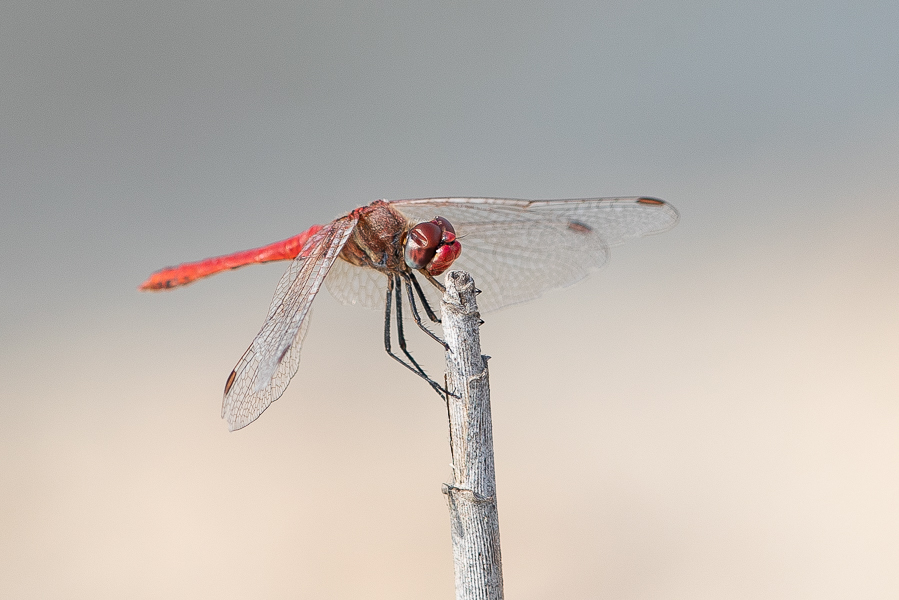This image is an extremely close-up shot of a dragonfly clinging to the top of a tall, reed-like twig, which is predominantly white with hints of gray and brown. The dragonfly's six black legs firmly grasp the twig's tip. The face of the dragonfly, shown in remarkable detail, features two large, bulbous red eyes, a small red nose, and a red jaw. The head and the first segment of its body are a dark reddish-brown to maroon color, while the rest of the thin, straight body extends out of focus in a bright reddish-orange hue. The wings are delicate and clear with noticeable veins running through them, adorned with a few brown spots along their edges. The background transitions smoothly from a light purple at the top to a pinkish-white hue near the bottom, creating a beautiful ombre effect that enhances the dragonfly's vivid coloration.